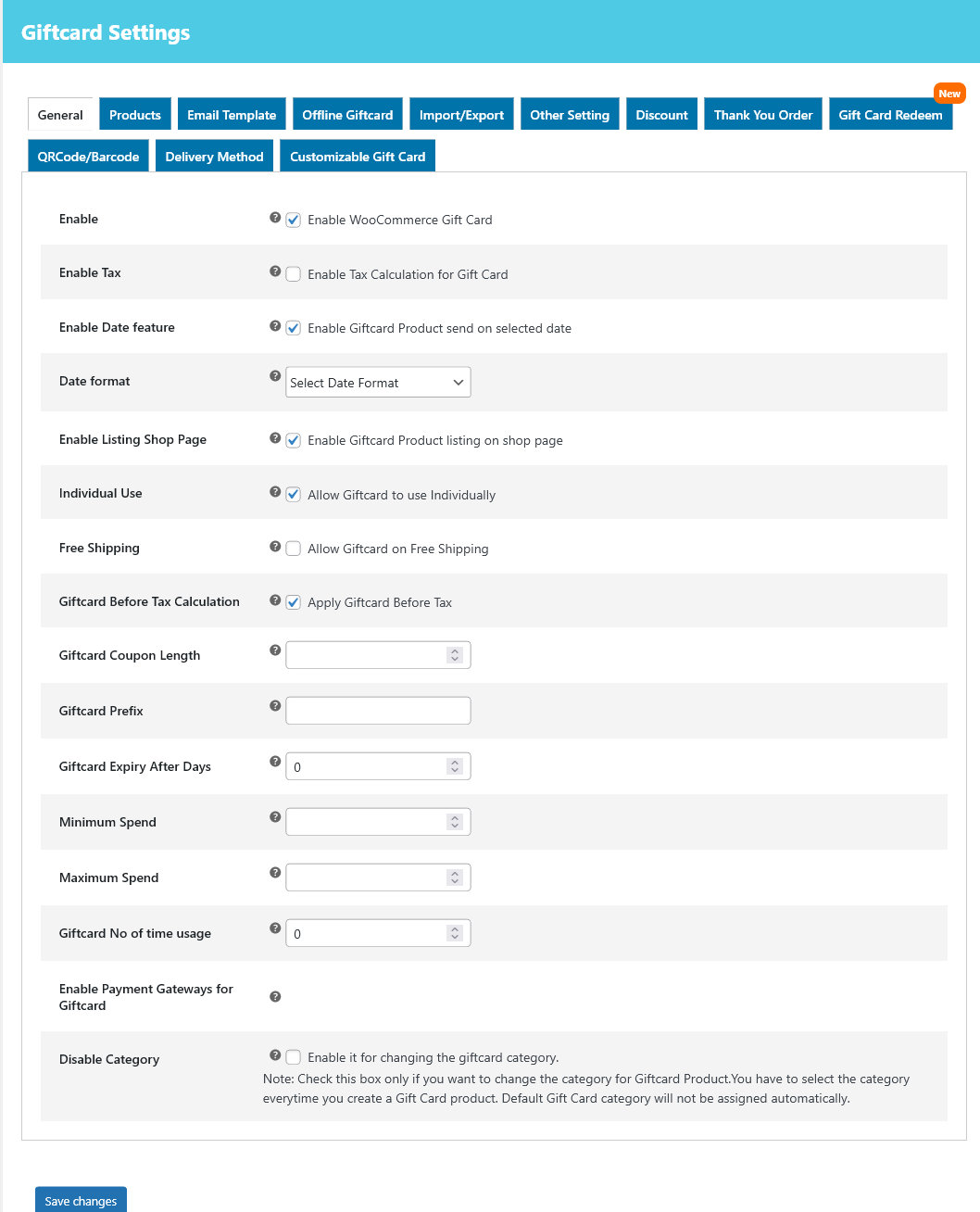In the settings panel with a light blue color scheme dedicated to configuring gift cards, the screen displays various sections and options. The main sections include General Settings, where you can configure productos, email templates, offline gift card options, import/export settings, and weather settings. 

Additional features include customizing discounts, thank you orders, and methods for redeeming gift cards. There are options like a driver card/broker configuration and the selection of delivery methods. The section also allows the addition of customizable gift card features including text enablement for bookmarks, data features, and gift card products.

Users can enable or disable various features such as digital use, free shipping, and tax-related applications. They can also define parameters like gift card length, prefix, expiry dates, and set minimum and maximum spends for each gift card.

Other advanced settings include enabling a payment gateway specific to gift cards and setting typical categories. The interface reassures “no tricks,” although it notes that creating a category for gift cards will require selecting and managing various subcategories. A blue bar at the bottom of the screen provides the option to “Save Changes.”